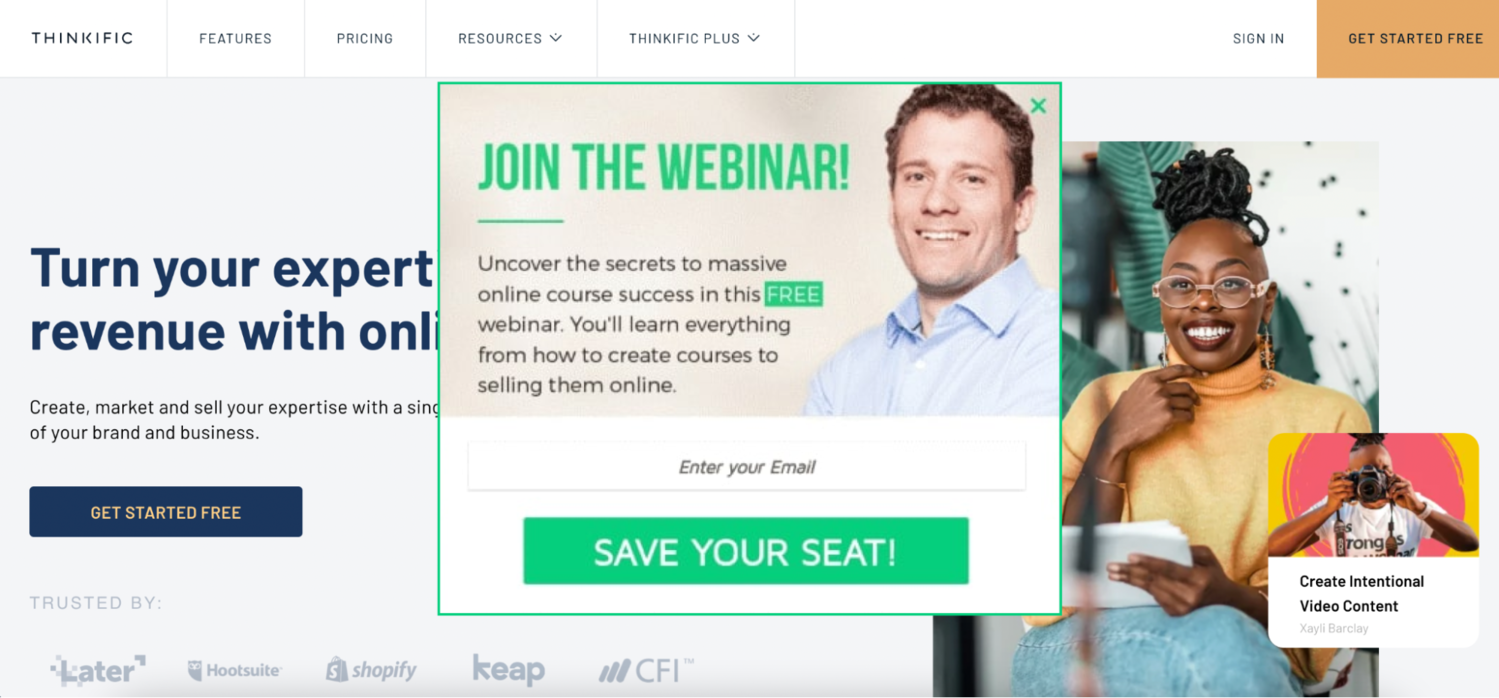The upper left corner of the image features the logo "Thinkific". Moving to the right, there are several navigational links labeled "Features," "Pricing," and "Resources," each accompanied by a pull-down menu icon. Further to the right, there is an option to "Sign In," and an orange button labeled "Get Started Free."

Beneath this header, the main text reads “Turn your expert knowledge into a profitable revenue stream” but is partially cut off. Below this text, there is an image of an African American woman with her hair styled in an updo. She is wearing glasses, a yellow turtleneck, and blue jeans.

A pop-up overlay appears on the left side of the image with the following text: "Join the webinar: Uncover the secrets to massive online course success in this FREE webinar. You'll learn everything from how to create courses to selling them online." The word "FREE" is highlighted inside a white rectangle, contrasting with the black font of the rest of the message. Below this text, there is a data field prompting users to "Enter your email," followed by a green button with white text that says "Save Your Seat." The entire pop-up is outlined in green with a green "X" in the upper right corner for closing the popup.

On the right side of the image, there is a photograph of a white man with dark hair wearing a blue shirt. The "Join the Webinar" text is prominently displayed in green, with a green line beneath it, while the rest of the text is in black font.